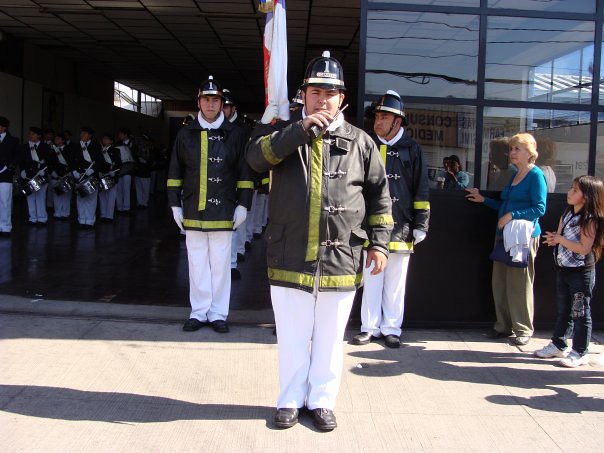Three gentlemen in striking uniforms stand prominently in the foreground, wearing black caps with white stripes and small white emblems at the top. Their attire resembles firefighter garb, featuring yellow jackets with distinctive black and yellow striping, held together by large clasps. Completing their uniforms are white pants and black shoes. The gentleman at the center appears to be communicating into a walkie-talkie. Flanking this central trio, to the right, is a woman clad in a blue shirt and tan pants, accompanied by a little girl dressed in black jeans and white shoes. In the background, extending to the left, there's a formation of individuals in similar uniforms, likely forming part of a marching band. This assembly is situated inside what appears to be a garage, evident from the glass windows and structural context, possibly reflecting the metallic instruments held by some members of the band. This scene, steeped in a formal yet ceremonially vibrant ambiance, underscores a context reminiscent of civic service personnel rather than purely military or civilian attire.